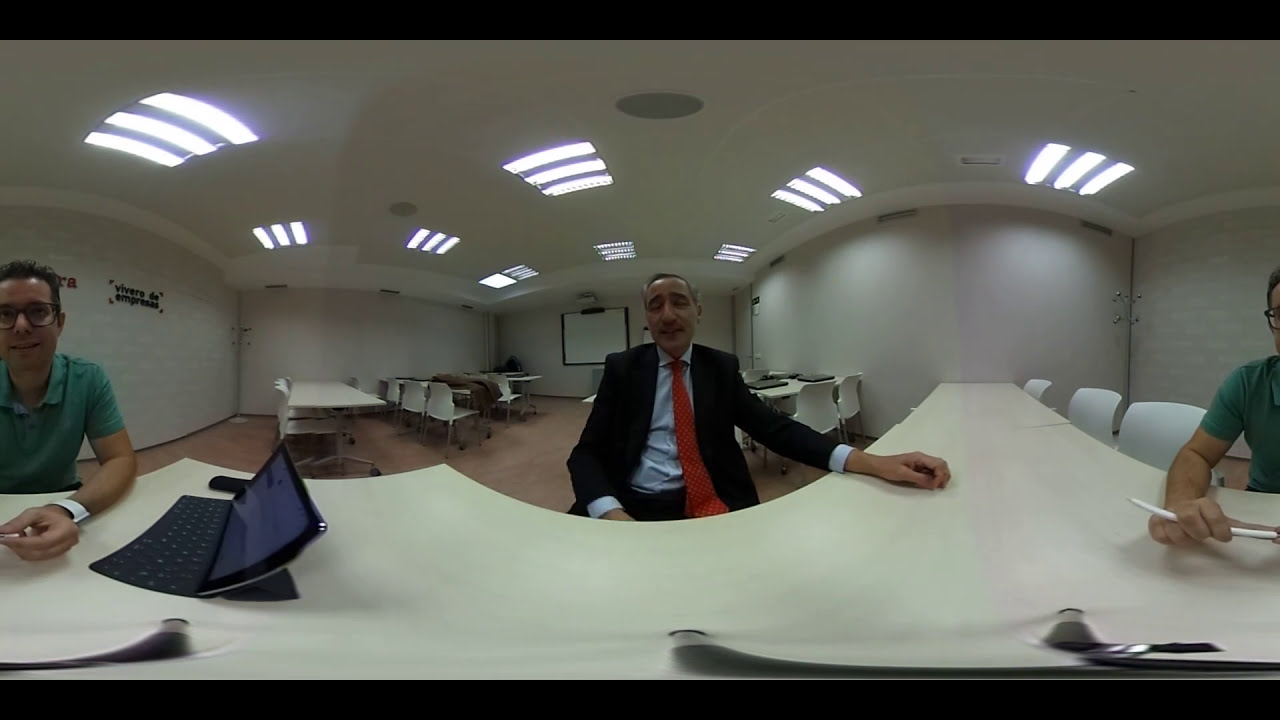In this indoor, office-like scene captured with a wide, convex lens, two men are the primary subjects. Central to the image is a man with gray hair and tan skin, possibly of Indian descent, who is seated behind a white table. He wears a black suit paired with a light blue button-up shirt and a red tie. His eyes appear droopy or closed, suggesting he might be blinking mid-conversation. In front of him, a laptop hints at his engaged activity, perhaps addressing the camera or another person.

To his left, part of another man is visible, wearing a green, short-sleeved polo shirt. He has short brown hair, black glasses, and a white watch, and he is holding a white pen. A distorted view of a tripod-like object in front of him suggests that the scene may be live-recorded or captured in an unconventional manner.

The setting includes several empty tables and office chairs in the background, contributing to a classroom or conference room-like atmosphere. A whiteboard adorns the back wall, under bright lighting, and the phrase "Viver de Impressus" is faintly visible on the wall, indicating a foreign language context.